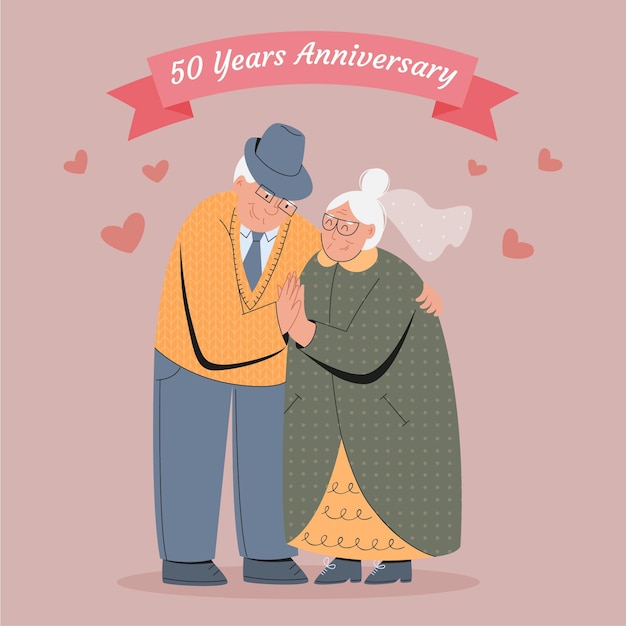The image is a digital rendering, perfect for a greeting card, celebrating a couple's 50th anniversary. At the center, an elderly couple in their 80s embraces lovingly. The man, slightly taller and standing on the left, has gray hair under a fedora, wears rectangular glasses, and is dressed in a yellow and orange cardigan over a shirt and tie, complemented by blue pants and dark gray shoes. His left arm extends over the woman's shoulder, and their opposite hands press together in a tender gesture. The woman, on his right, has her white hair in a bun and sports glasses as well. She wears a green jacket with a yellow collar and an accompanying yellow dress.

Above them, a pink, symmetrically arched ribbon features elegant white cursive text reading "50 years anniversary." The background is a soft grayish-mauve, accentuating the simplicity and warmth of the scene. Scattered hearts enhance the celebratory feel, with three small hearts adorning each side of the couple. The overall palette includes shades of green, yellow, blue, white, pink, red, and a peachy undertone, making the illustration vibrant yet harmonious. This touching image beautifully encapsulates a milestone of love and commitment, making it an ideal design for an anniversary card.